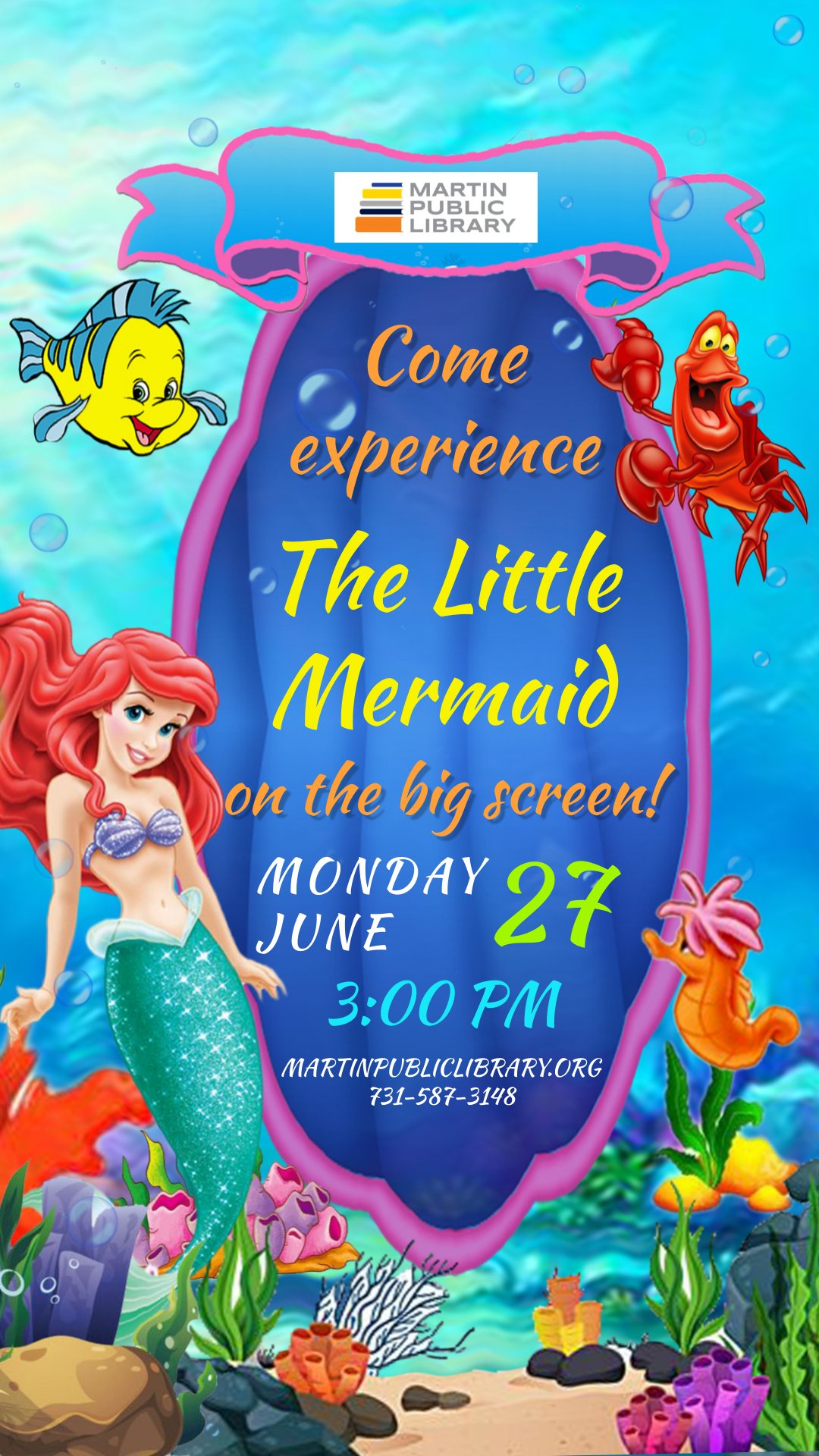This vertical advertisement scan features vibrant characters from Disney's The Little Mermaid set against an enchanting underwater backdrop. In the top left, the cheerful Flander is depicted in his iconic blue and yellow hues, while to the right, Sebastian stands out in vivid red. Ariel, with her flowing red hair and characteristic blue and purple mermaid outfit, is positioned towards the bottom left, next to a curious orange seahorse. The scene is set against a lively backdrop of corals below and shimmering water above.

Prominently displayed in the center is the Martin Public Library logo in gray and white. Beneath the logo, colorful text invites viewers to "Come experience The Little Mermaid on the big screen." The event details are creatively highlighted: "Come experience" is in orange, "The Little Mermaid" in yellow, and "on the big screen" returns to orange. Details continue with "Monday" and "June" in white, "27" in green, and "3 p.m." in blue.

Additionally, at the bottom are the contact details: "martinpubliclibrary.org" and "731-587-3148," ensuring that all necessary information is clearly presented. This detailed and vividly colored advertisement perfectly captures the magic and allure of The Little Mermaid, inviting all to a special screening on Monday, June 27, at 3 p.m.